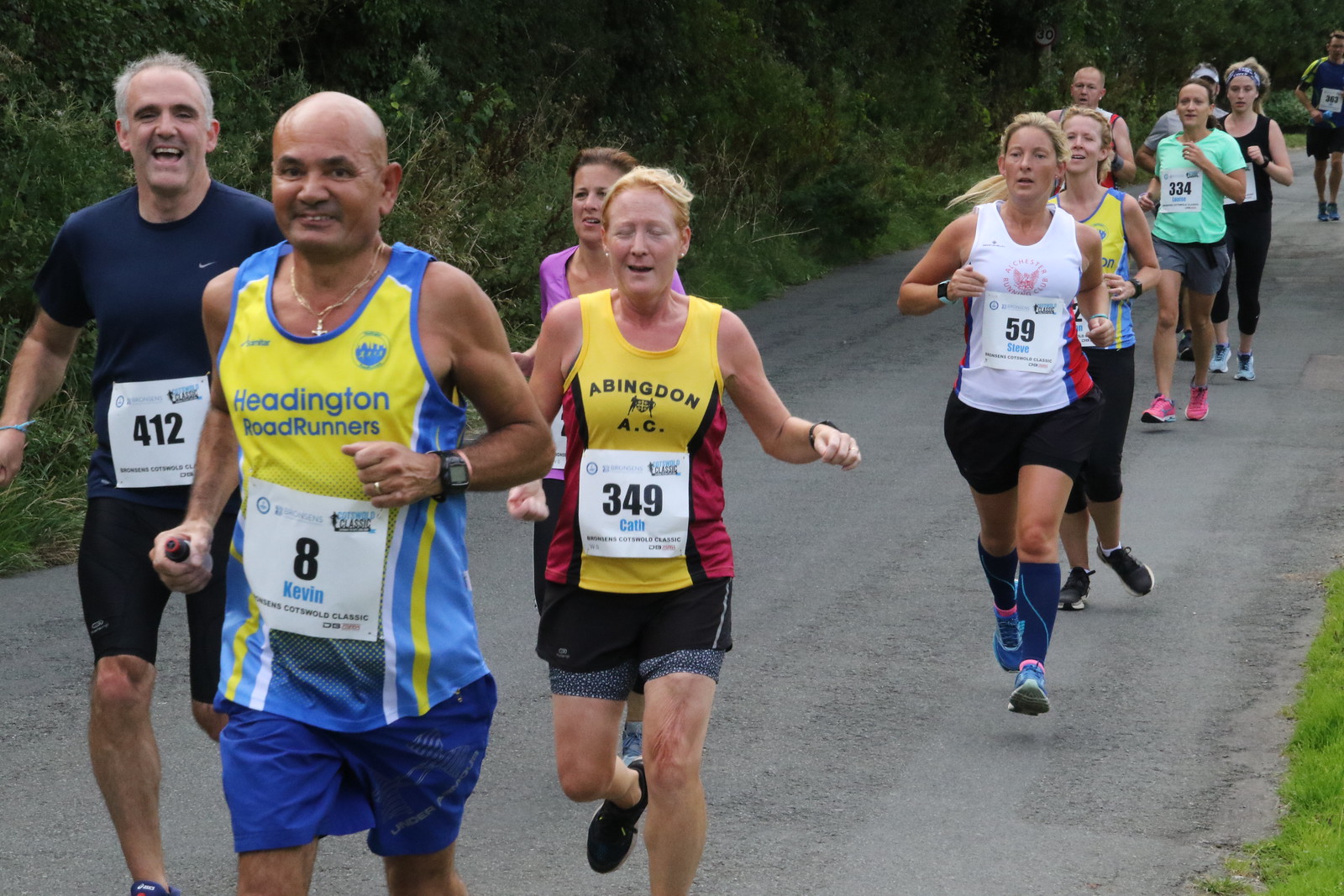This color photograph captures an invigorating scene of a countryside race with a group of about 11 runners on a small, paved road that lacks line markings. The road is flanked by lush green grass on the right and a backdrop of shrubs, bushes, and small trees on the left, giving it a serene, natural setting. Prominent in the foreground is a bald man in his 40s, wearing a yellow and blue striped tank top, blue shorts, and a black wristwatch, identified by the race number 8 and the name Kevin on his shirt. He runs with a smile and appears to be in motion. Just behind Kevin, slightly to the left, is an older man with gray hair donning a black tank top and shorts, marked with the number 412. This man is also smiling, adding a lively atmosphere to the race.

To Kevin’s right runs an older blonde woman in a yellow tank top with red sides and black shorts, branded with the race number 349 and the name Cath. She is in motion, her arms out at her sides, though her eyes are closed. Slightly behind her, to the left, is a younger woman in a pink top, though only her shoulder and head are visible. Another notable participant is a younger blonde woman in a white tank top and black shorts, sporting the race number 59. She runs with both feet off the ground, navy blue knee socks, and blue tennis shoes, adding dynamism to the scene.

Further back, a woman in a yellow tank top and black shorts appears partially visible, her race number obscured. Trailed by these runners is another woman, distinguishable by her turquoise blue t-shirt, gray shorts, pink tennis shoes, and the race number 334. Her gray-haired, older gentleman companion appears beside her, both seemingly walking briskly. In the distance, the figures of several more runners blur into the background, with one being a woman in longer black sweatpants and a black tank top. The farthest individual is a man, whose details are too indistinct to discern.

This detailed depiction showcases diverse runners in various competitive and enthusiastic expressions, set against a tranquil countryside backdrop, perfectly capturing the essence and energy of the race.